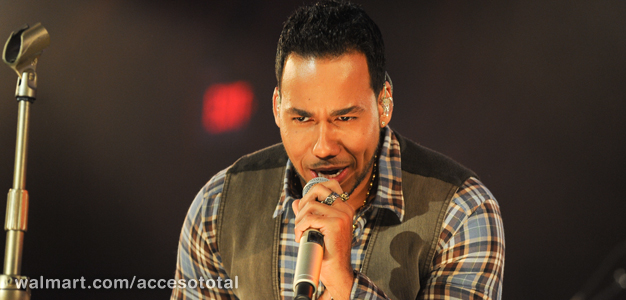This rectangular photograph features a man performing on stage against a dark, hazy background. To the left, a blurry red light, possibly an exit sign, is visible. The man, with light brown skin and short dark hair, has an earpiece in both ears and is holding a microphone to his lips with his left hand. He is dressed in a blue and black plaid button-down shirt underneath a denim vest, and wears silver rings on his right index and middle fingers. A silver-and-black microphone stand is positioned to the left of him in the image. At the bottom left corner of the image, the words "walmart.com/access" are displayed in white letters.